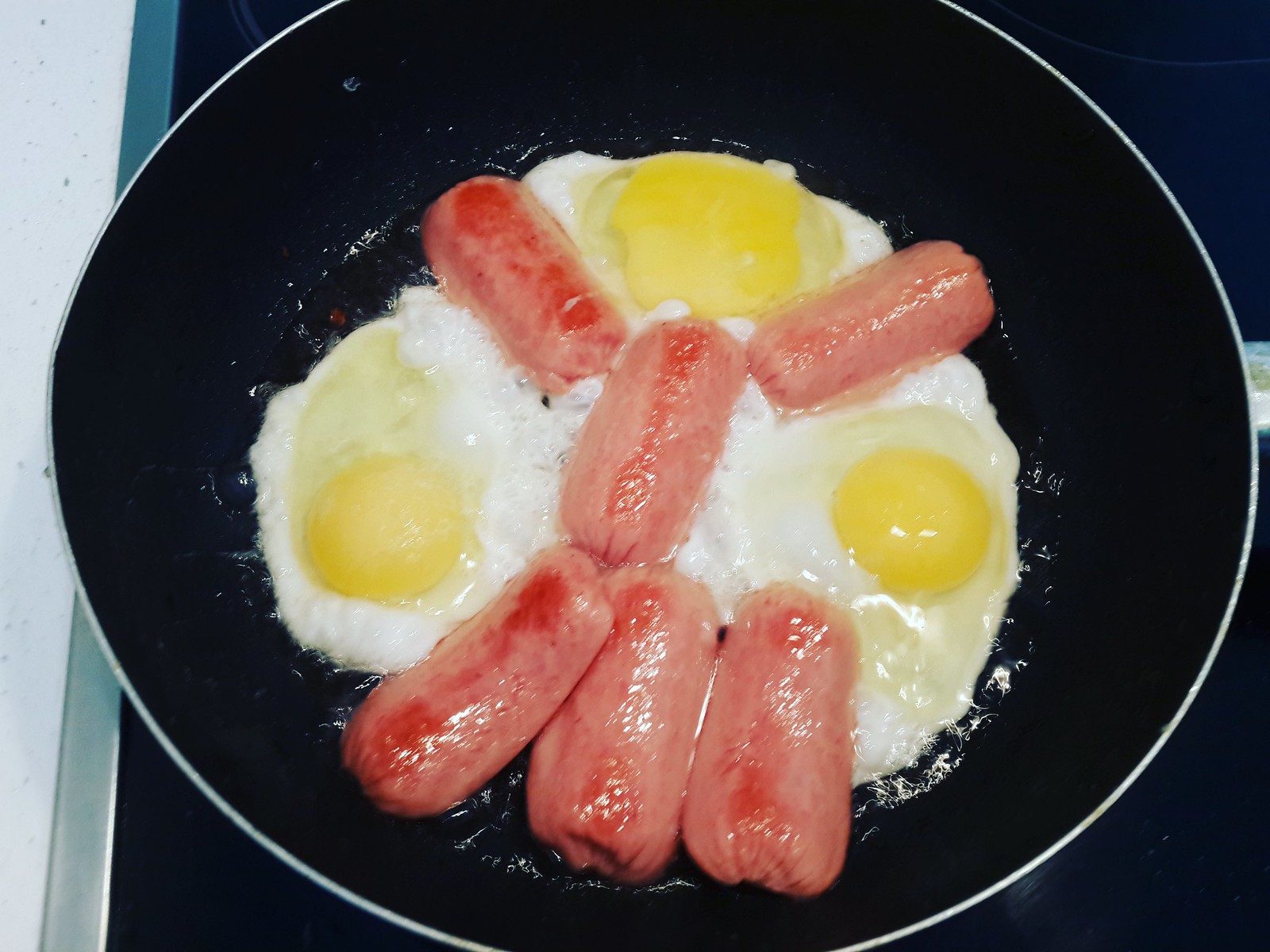This color photograph captures a low-quality image, likely taken with a phone camera, of breakfast being cooked in a black non-stick frying pan on an induction cooktop. Three eggs are positioned at 12 o'clock, 3 o'clock, and 9 o'clock, their yolks still soft and translucent as the whites begin to solidify. Scattered between the eggs are six thumb-sized sausages or mini hot dogs, pinkish in color and starting to turn dark red on the tops. Three sausages align along the bottom of the pan, while one in the center forms a Y shape, effectively separating the eggs. The sizzling oil bubbles around the edges of the food. Visible on the far left edge is a modest white linoleum countertop, adding context to the kitchen setting. The scene is devoid of additional items, people, animals, or ornate details, focusing entirely on the cooking process.